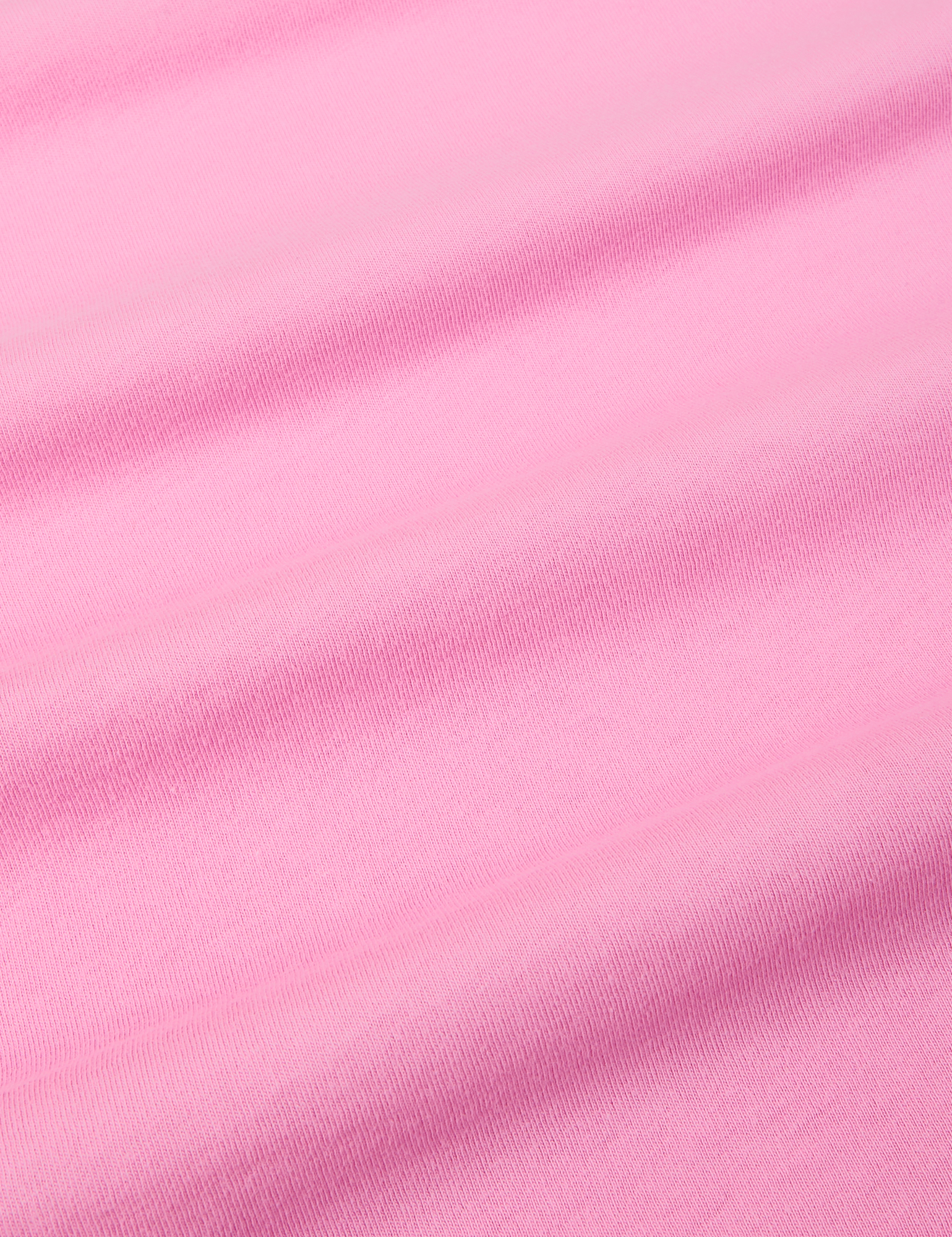This image presents a detailed, up-close view of a light pink fabric swatch, characterized by its fine knit texture. The fabric appears wavy, with about three to four raised ripples creating subtle shadows and making areas of the fabric slightly darker pink. The light bubblegum pink material is shown in a zoomed-in perspective, allowing the visibility of individual threads. Overall, the image focuses solely on the intricate details of the fabric's texture and color, devoid of any text, numbers, or other elements.